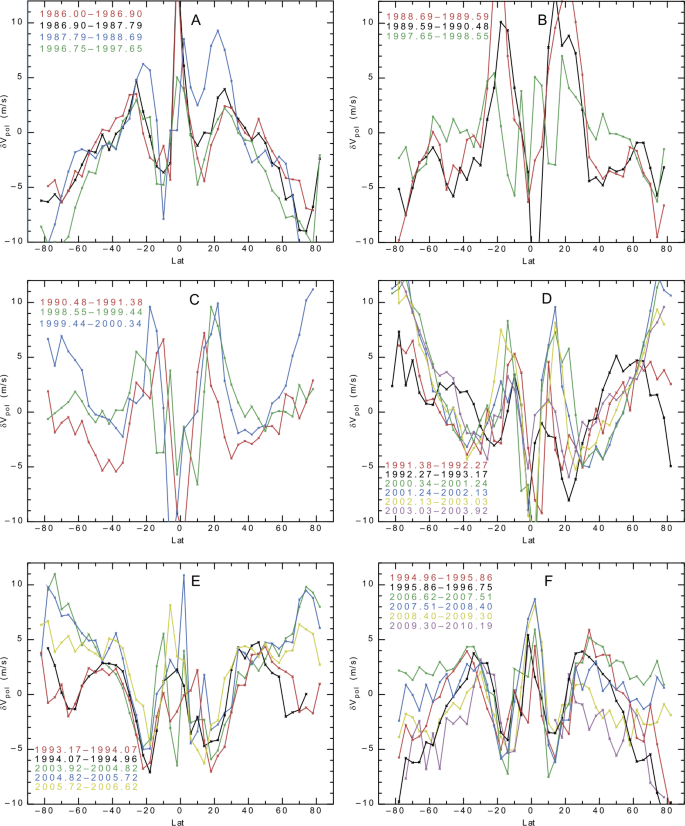The image displays a set of six graphs labeled A through F, each illustrating data with lines in various colors including red, blue, yellow, black, and green. These graphs chart fluctuations over a range of years, depicted along the x-axis, which is labeled "lat," indicating latitude with values spanning approximately -80 to 80. The y-axis is noted as "sigma v subscript pol m/s," ranging from -10 to 10. The graphs are plotted on a white background, making the colorful but jagged lines—representing different years—stand out. However, the lack of further descriptive signage or context renders it challenging to interpret the meaning behind the visual data. Notably, graphs A, B, and C feature more widely spaced lines, making them easier to distinguish, while the lines in graphs D, E, and F are densely packed, complicating visual differentiation.